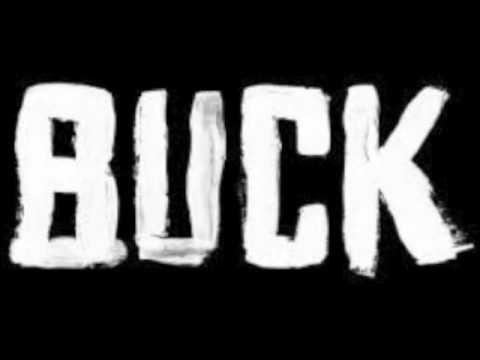The image is stark and simple, featuring a solid black background with large, white, all-capital letters spelling out "B-U-C-K" across the center. These blocky letters stretch horizontally from left to right, occupying approximately two-thirds of the total space and leaving a small margin above and below them. The lettering appears hand-painted, with uneven edges and noticeable smudging, particularly on the bottom right leg of the "K" and along the sides of various letters, giving the impression of graffiti. The lack of curvature in the characters adds to the rough, almost sloppy aesthetic, suggesting that the text was drawn by hand rather than using a precise text tool. The white paint has shaded areas which, combined with the black background, create a faint grayish hue in some spots, further emphasizing the textured, imperfect nature of the image.